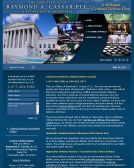The image depicts a destination landing page with a predominantly blue background. Spanning the top of the page is a blue rectangular banner featuring white text. Below this banner sits an image of a grand, white marble building reminiscent of historic landmarks like a courthouse or the Parthenon, complete with seven columns that stretch across its facade.

On the right side of the page, there are three distinct, curved images. Beneath these curves, a lighter blue rectangular banner also hosts white text. Further down, the page is organized into informational paragraphs. Each paragraph is prefaced by a yellow header, followed by detailed content in white text. There appear to be approximately four paragraphs in total.

Interspersed in the middle section of the page, both to the right and left, are pockets of white text. Adjacent to these text blocks are vertically stacked rectangles that are a lighter shade of blue compared to the background. The layout is cohesive, providing a structured visual hierarchy for visitors.